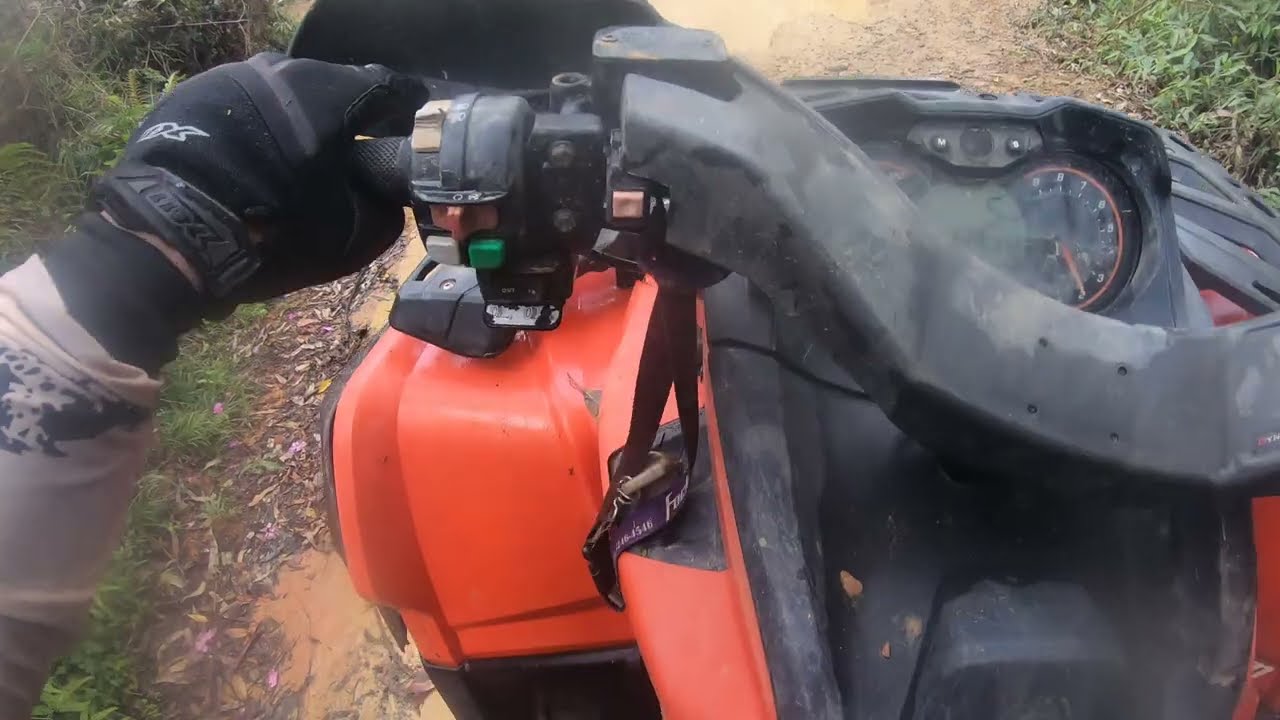This photograph, captured from a GoPro mounted on a helmet, offers a rider’s-eye view of an off-road vehicle, possibly a dirt bike or ATV. The primary focus of the image is the vehicle itself, which features a striking combination of black, gray, and bright orange colors. The rider’s left hand, clad in a black glove and a black and white long-sleeved shirt, firmly grips the throttle. The handlebars, turned to the right, reveal a black control panel that includes two readouts. Below, the front left wheel is visible, suggesting the vehicle type. The scene is set on a light brown dirt path, flanked by a mix of green vegetation and some dead flowers and leaves. The clarity of the grass and foliage indicates that the vehicle is stationary. It appears to be a clear, daylight moment, providing a vivid snapshot of this outdoor adventure.